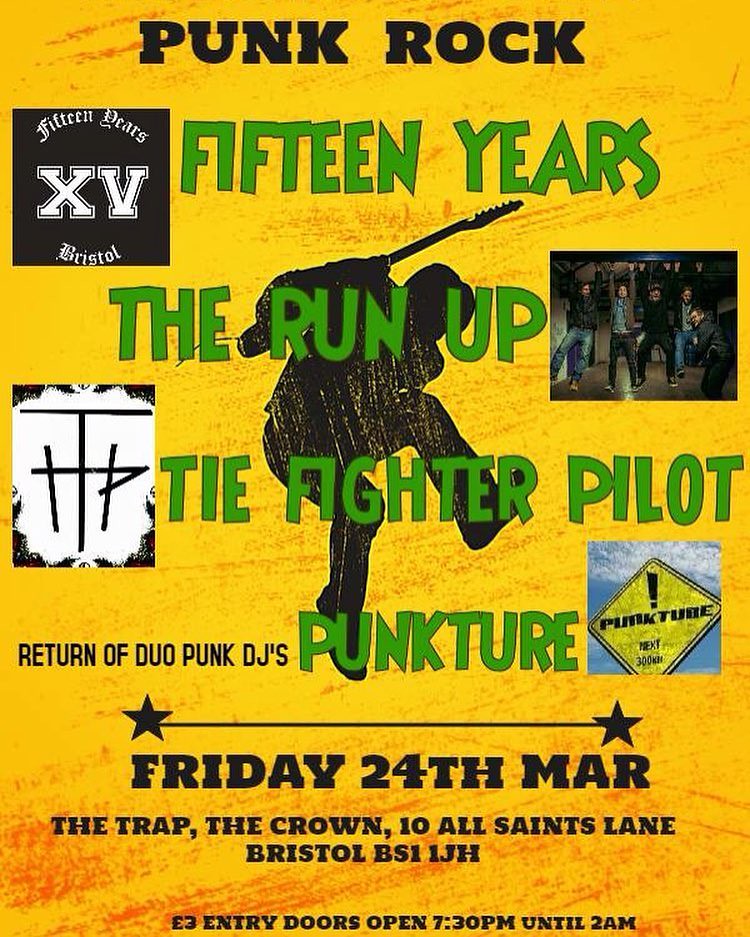This vibrant flyer is an advertisement for a punk rock event featuring multiple acts, celebrating "15 Years." Dominated by shades of yellow and orange, it prominently showcases a silhouette of a guitarist. "Punk Rock" is emblazoned across the top in black text, followed by other green texts: "15 Years," "The Run-Up," "Thai Fighter Pilot," and "Return of Duo Punk DJs Puncture."

To the left, there's a black square stating "15 Years XV Bristol," and to the right of "The Run-Up," an image shows four people running towards a stage. Next to "Puncture" is a yellow diamond-shaped sign with an exclamation mark, reading "Puncture next 300 km."

The flyer also features various images, including the band members hanging onto a railing and a "Puncture" warning sign. It notes details of the event: "Friday, 24th March, The Trap, the Crown, 10 All Saints Lane, Bristol." Entry doors open at 7:30 PM and the event continues until 2 AM, with an entrance fee of three British pounds.